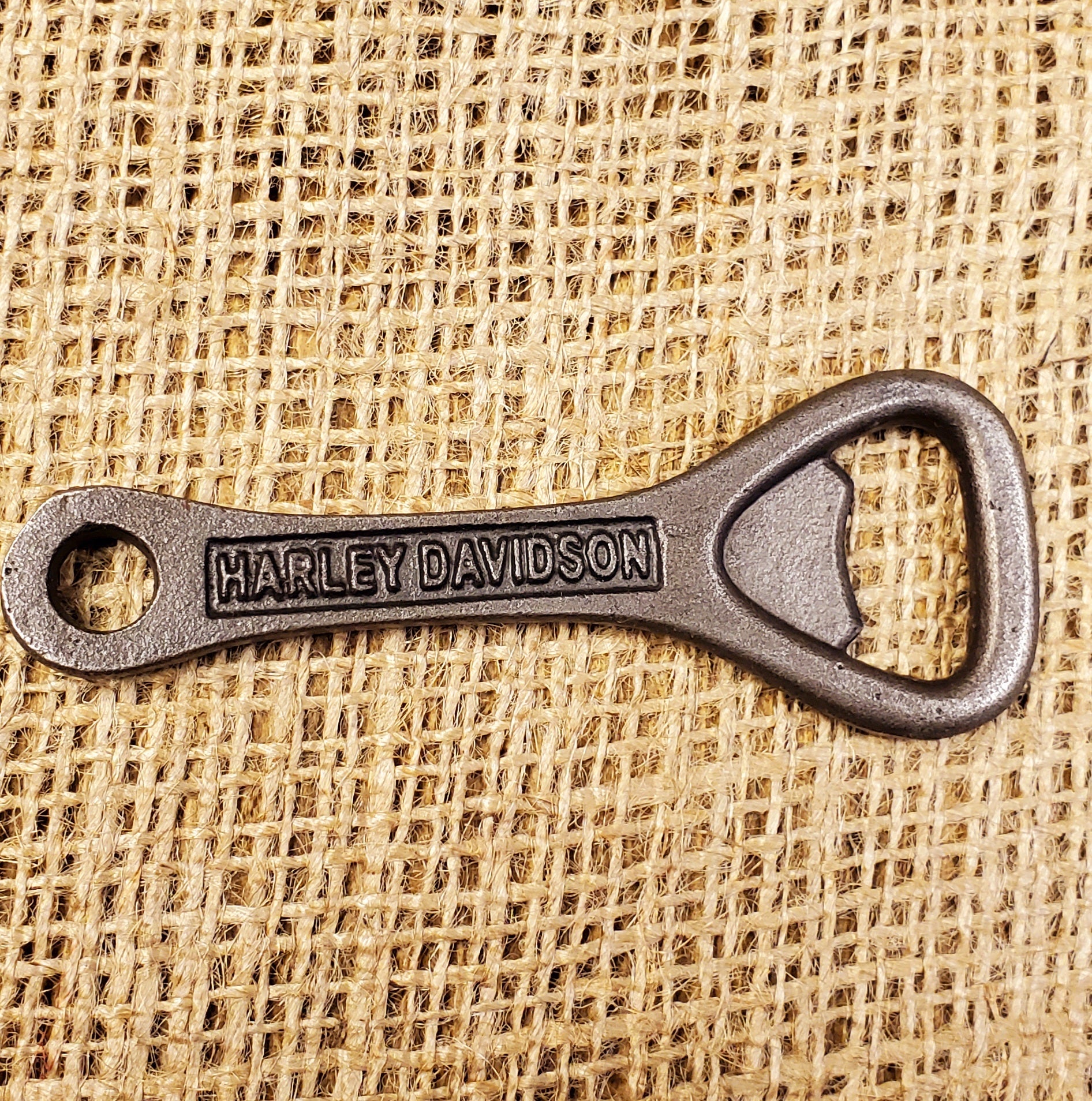The photograph showcases a Harley-Davidson branded bottle opener made of dark gray metal, prominently displayed in the center of the image. The metal tool has rounded edges and features a small hole at one end, possibly for attaching to a key ring. The bottle opener is stamped with the words "Harley-Davidson" across its middle, signifying its association with the iconic motorcycle brand. It rests atop a woven mat made of straw or burlap, which is a beige or cream tan color, providing a contrasting backdrop that highlights the dark, sturdy appearance of the bottle opener.